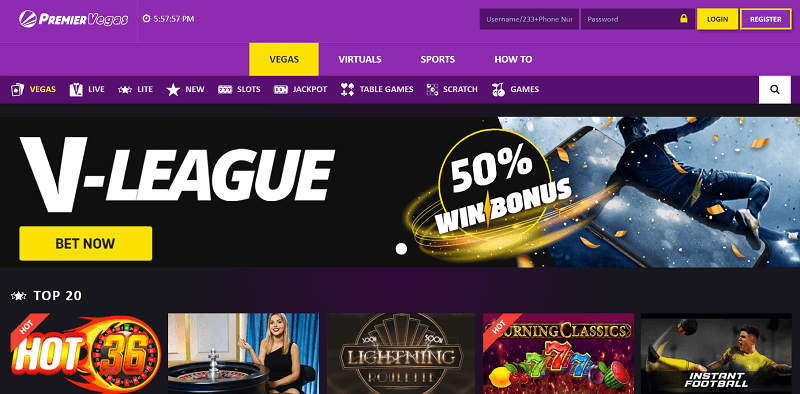This is a detailed description of the Premiere Vegas website at 5:57 PM:

The website, titled "Premiere Vegas," features a prominent purple band across the top. On the upper left corner, the site's name "Premiere Vegas" is displayed. The current time is shown as 5:57 PM.

On the upper right corner, there is a user interface element for logging in, which includes fields for "Username," "Phone Number," a secured "Password" indicated by a lock icon, and buttons for "Login" and "Register."

Below the purple band, the navigation menu is visible with several tabs. The first tab is labeled "Vegas" in black. Other tabs include "Virtuals" and "Sports" in white text and the tab "How to" also in white, placed on purple backgrounds. Another "Vegas" tab is highlighted in yellow.

Further navigation options include "Live" shown twice in white text, "New Slots," "Jackpot," "Table Games," "Scratch Games," and a second "Live" option.

On the right side of the top navigation bar, there is a search icon represented by a magnifying glass in a white button with black font.

Below the navigation bar, there is a banner featuring a yellow button with black text that reads “Bet Now,” promoting a V League 50% win bonus. The banner visually showcases a man dancing, surrounded by floating imagery of money, including what seems to be dollar bills and gold coins.